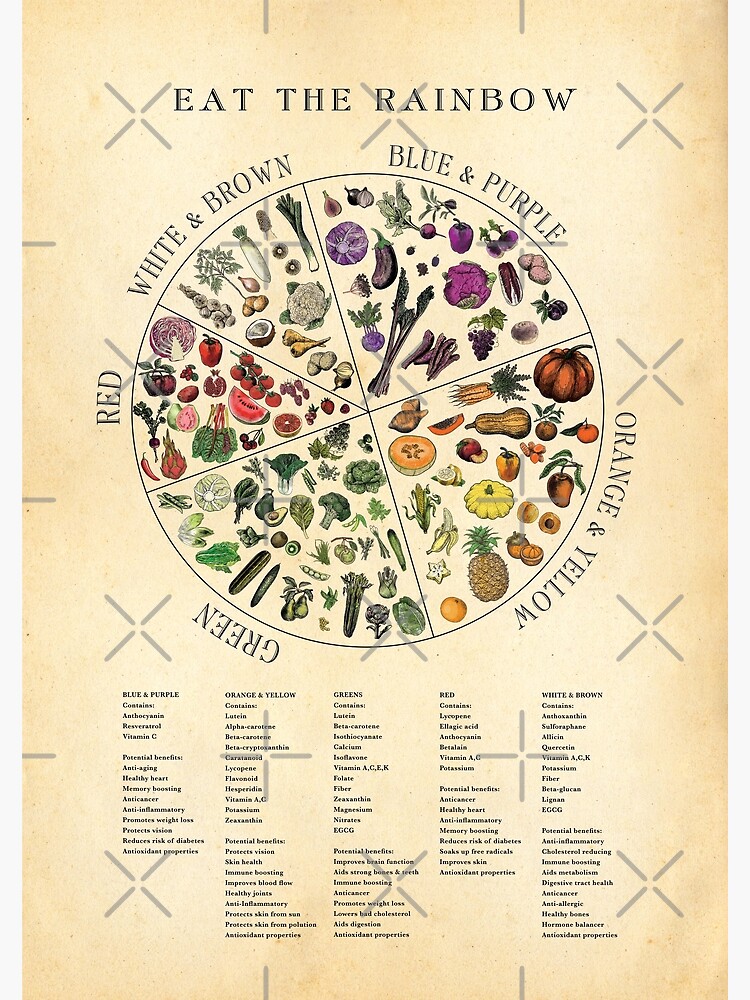This is an illustration titled "Eat the Rainbow" at the top in bold, black capital letters. It features a detailed pie chart divided into five color-coded sections, each representing different categories of foods. The blue and purple section includes red cabbage, turnips, beets, and shallots. The orange and yellow section showcases foods like oranges, pineapple, cantaloupe, pumpkin, squash, and carrots. The green section is packed with celery, peas, kiwi, avocados, cabbage, cucumbers, and lettuce. The red section contains watermelon, rhubarb, red cabbage, tomatoes, and grapefruit. Finally, the white and brown section features coconuts, leeks, and cauliflower. The entire pie chart is set against a backdrop adorned with small silver X's for a textured design. At the bottom of the image, there are five columns listing all the foods shown in the chart along with their potential benefits, although the text is very small and difficult to read.